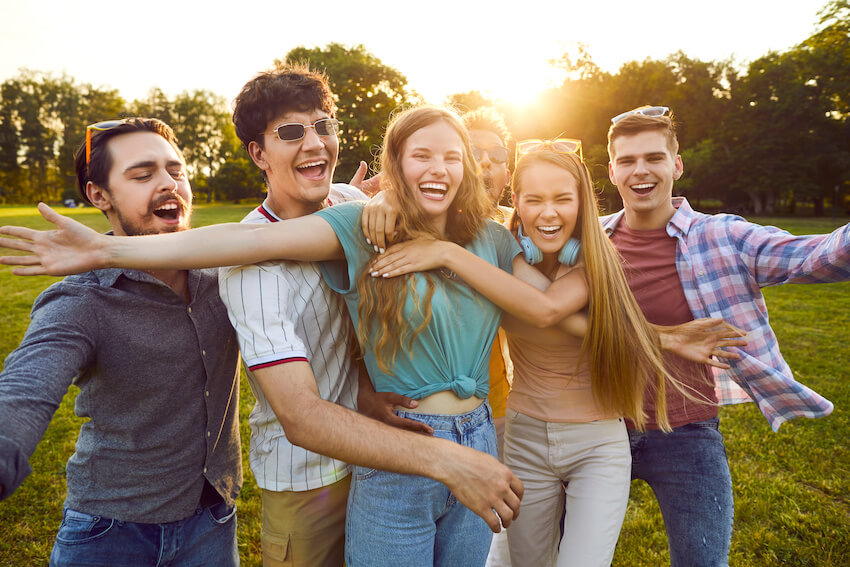This is a horizontal rectangular photograph depicting six friends—four men and two women—posing with their arms spread out in an outdoor setting. They are all smiling and looking directly at the camera, standing on a grassy area with trees and bright sunlight in the background.

From left to right, the first man is dressed in a blue long-sleeved shirt with jeans, and he has sunglasses on his head. Next to him, another man with brown hair is wearing a white short-sleeved shirt and khaki pants, also with sunglasses. In the center, the woman on the left has long brown hair, a teal colored blouse tied around her waist exposing her midriff, and blue jeans. The second woman, also with long brown hair and sunglasses on her head, is wearing a coral top and beige pants. To her right, another man is dressed in a maroon t-shirt under a pink and blue plaid shirt, paired with blue jeans. Lastly, partially visible behind the group, there is someone wearing sunglasses.

The scene is filled with a sense of camaraderie and joy, emphasized by the casual attire and relaxed poses of the friends.